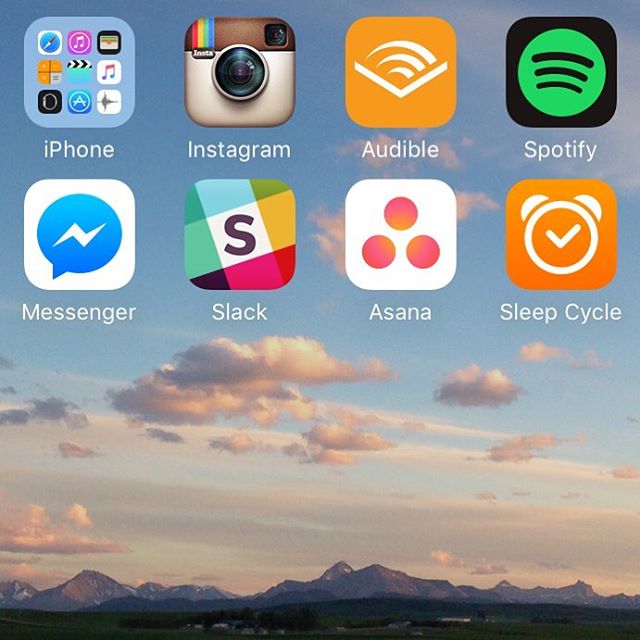**Detailed Caption:**

The image depicts a smartphone app screen set against a scenic mountain background at the bottom. The screen is divided into panels, with the top panel being brown and the bottom panel beige. The mountain range at the lower part of the screen provides a rugged, natural backdrop.

At the top left corner, within a folder, a variety of iPhone apps are displayed. Notable app icons include:

- **Instagram:** Positioned centrally in the folder, featuring the classic camera logo.
- **Audible:** Displayed as an open book icon in white.
- **Spotify:** Represented by a green circle containing three black horizontal bars, all set against a black background.
- **Messenger:** Located at the bottom left, identified by a speech bubble with a white lightning bolt inside.
- **Slack:** Featuring a stylized 'S' formed by intersecting rainbow-colored squares.
- **Asana:** Displayed as a simplistic icon with three red dots set on a white background.
- **SleepSlego:** Depicted with a clock icon adorned with a white checkmark.

The descriptive elements of the application screen effectively combine vibrant app logos with a picturesque mountainous scene, creating an engaging visual contrast.